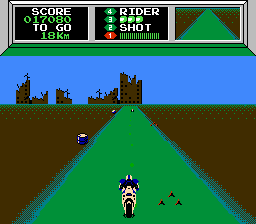A nostalgic screenshot captures the essence of a mid to late 1980s retro motorcycle racing game, likely from the NES era. At the heart of the scene, a motorcyclist is prominently centered, racing along a vivid green road. The periphery is marked by brown dirt delineating the out-of-bounds area. At the top of the screen, an informative menu displays critical information: "Score: 17,080," "To Go: 18 kilometers," and a selection of options labeled "4-3-2-1." Additionally, it indicates "Rider 3" and features three small ball icons, a "Shot" option, and what appears to be an energy bar. This intricately detailed snapshot harks back to a beloved era of classic arcade racing games.